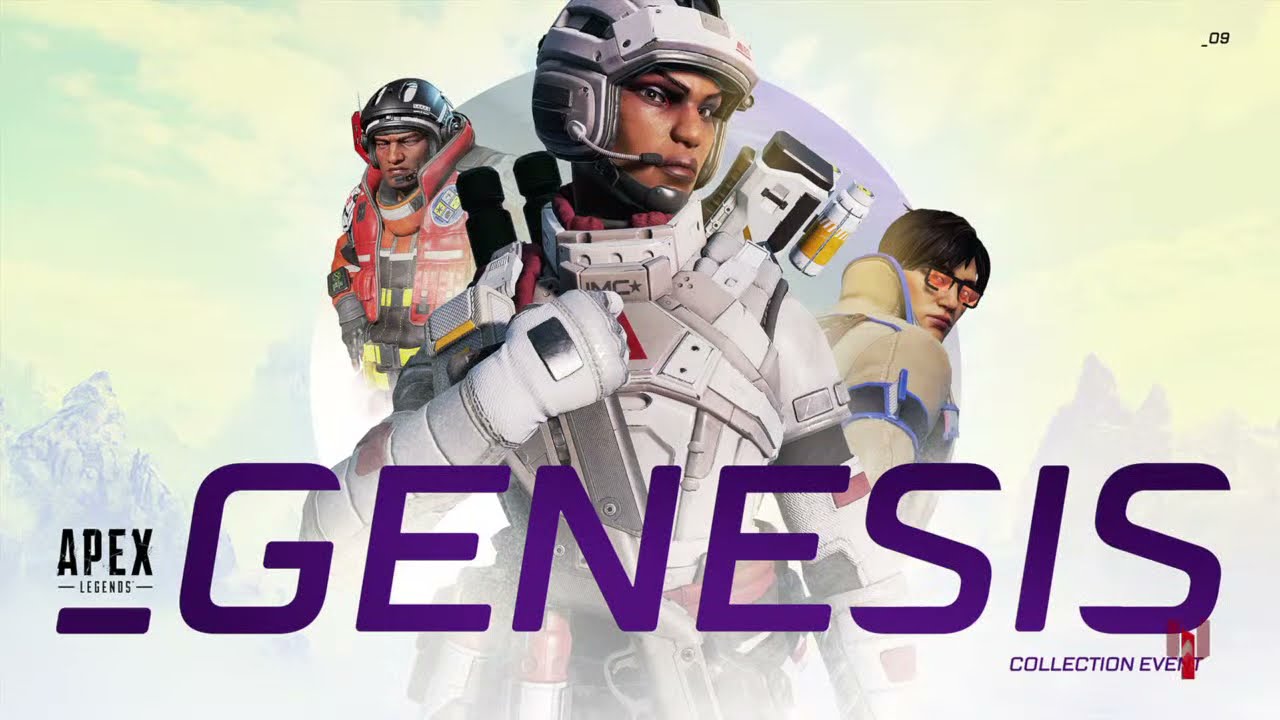The image is a detailed advertisement for a "Genesis Collection Event" in the video game Apex Legends. Dominating the image are large, italicized purple letters spelling "Genesis," with the words "Apex Legends" to the left in smaller print and "Collection Event" in blue at the bottom right corner, followed by "09" at the top right. The background showcases a fantastical scene featuring purple mountains under a greenish-yellow sky, and a blue planet further emphasizing the game's sci-fi setting.

In the foreground are three distinct characters. Centered in the image is a man in a white suit reminiscent of spaceman attire, complete with black, gray, and white canisters adorning his outfit. To his left stands another man in an elaborate red, orange, and gray soldier outfit, topped with a black helmet and featuring yellow accents. On the right, an Asian man with brown hair dons orange glasses and a beige jacket, offset by additional blue, white, and black details on his attire. A purple geometric shape, potentially a square or circle, is situated behind them, adding to the vibrant color scheme and futuristic theme.